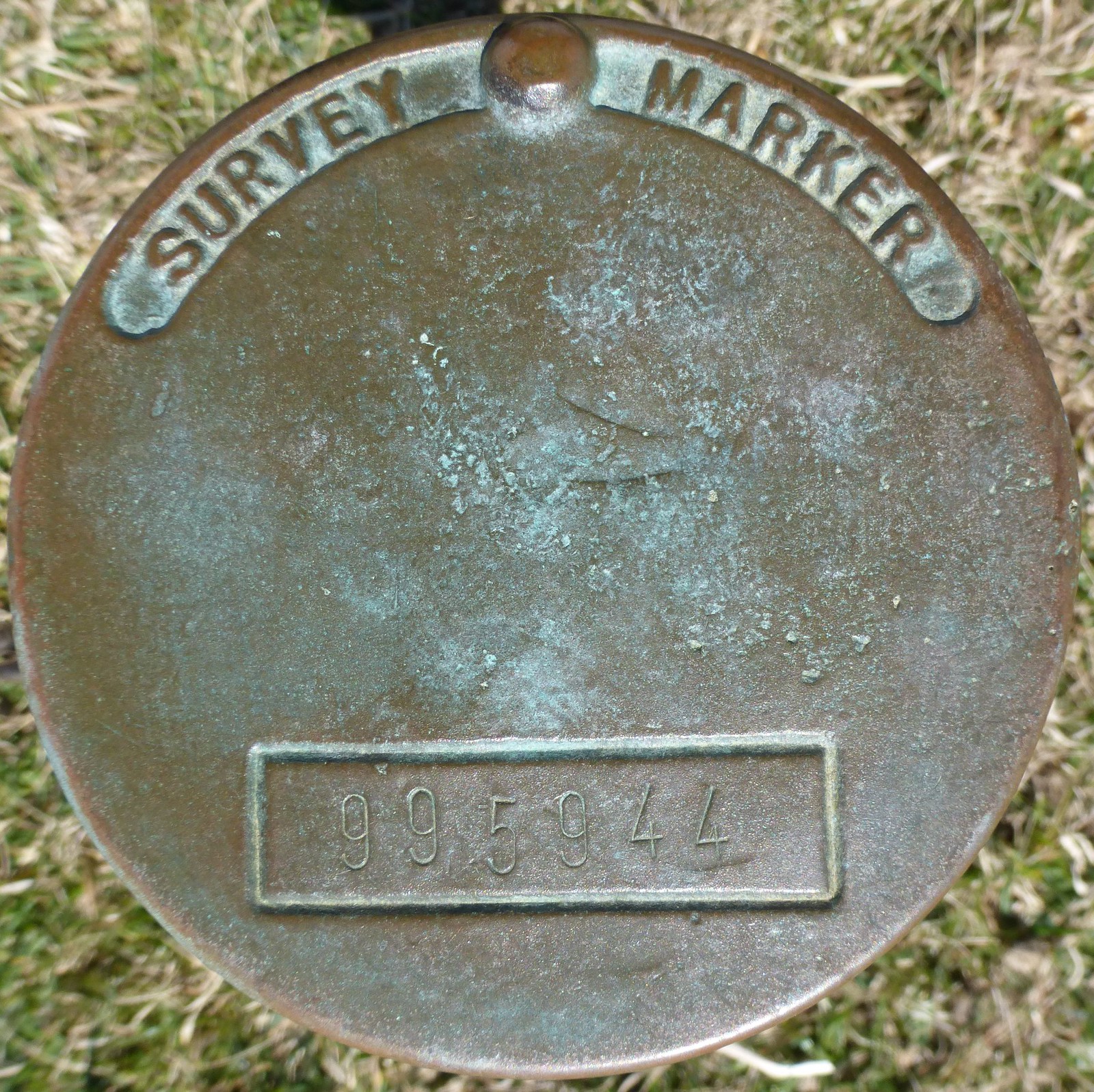The image displays a weathered circular survey marker, likely made of metal such as copper, given its green and brown patina indicating significant aging. The marker is set against a blurred backdrop of dried grass, which only peeks through at the corners, as the marker itself occupies most of the frame. Along the top curve of the marker, the words "Survey Marker" are prominently etched in a lighter arc. The surface shows signs of aging with white specks scattered across it, and there is a notable hole between the words "Survey" and "Marker." Towards the bottom of the circle, an engraved rectangle contains the numbers "995944," with some digits slightly misaligned, displaying an uneven stamping.